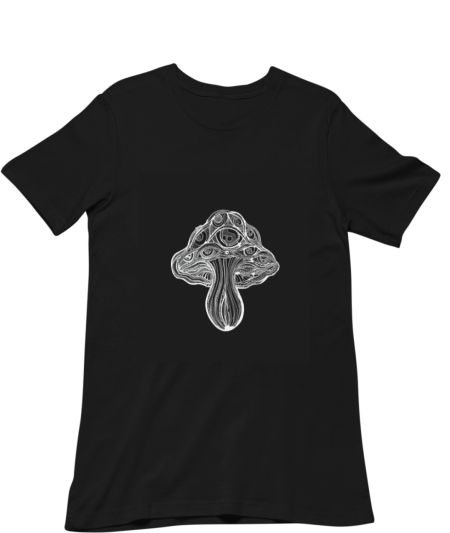This product image features a black t-shirt lying flat on a pure white background. The t-shirt displays a central, abstract, black and white illustration of a mushroom, occupying the center chest area. The mushroom's cap is ornate, adorned with swirling patterns and possibly intricate shapes resembling eyes or bubbles, giving it a psychedelic appearance. The stem of the mushroom is bulbous, extending downward in a manner reminiscent of a jellyfish. This detailed and abstract design contrasts starkly against the plain black fabric of the shirt, which has no additional text or markings. The sleeves extend outward to the sides, and the neckline forms a semi-circle at the top, emphasizing the clean, minimalist presentation likely intended for a product listing.